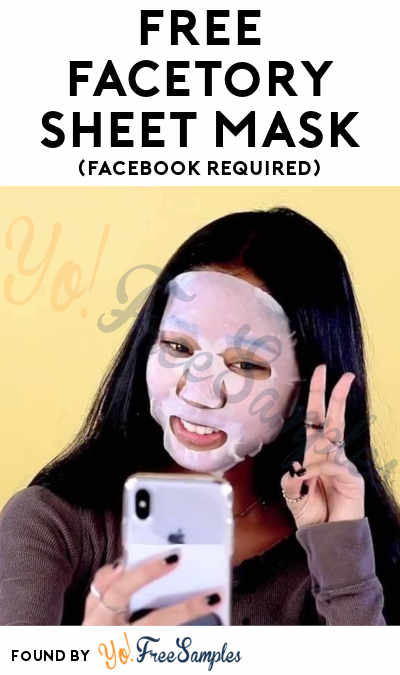The advertisement showcases a vertical photograph of an African American woman using a face mask, possibly for spa or beauty treatment. She has a darker skin tone with unusual, possibly photoshopped, white hands. Her black hair and black fingernails are easily noticeable, and she is adorned with rings on two fingers. The woman is dressed in a gray sweater and exudes a casual, relaxed vibe. She is taking a selfie with her silver iPhone while holding up a peace sign with her left hand. The background is yellow, adding a vibrant contrast to the overall image. At the top of the advertisement, in bold black all-caps, it reads "FREE FACETREE SHEET MASK," followed by a smaller text in parentheses stating "Facebook required." Below the photo, in a mix of yellow and blue cursive text, it says "found by Yo Free Samples." The overall style of the image suggests a social media advertisement aimed at promoting the beauty mask.